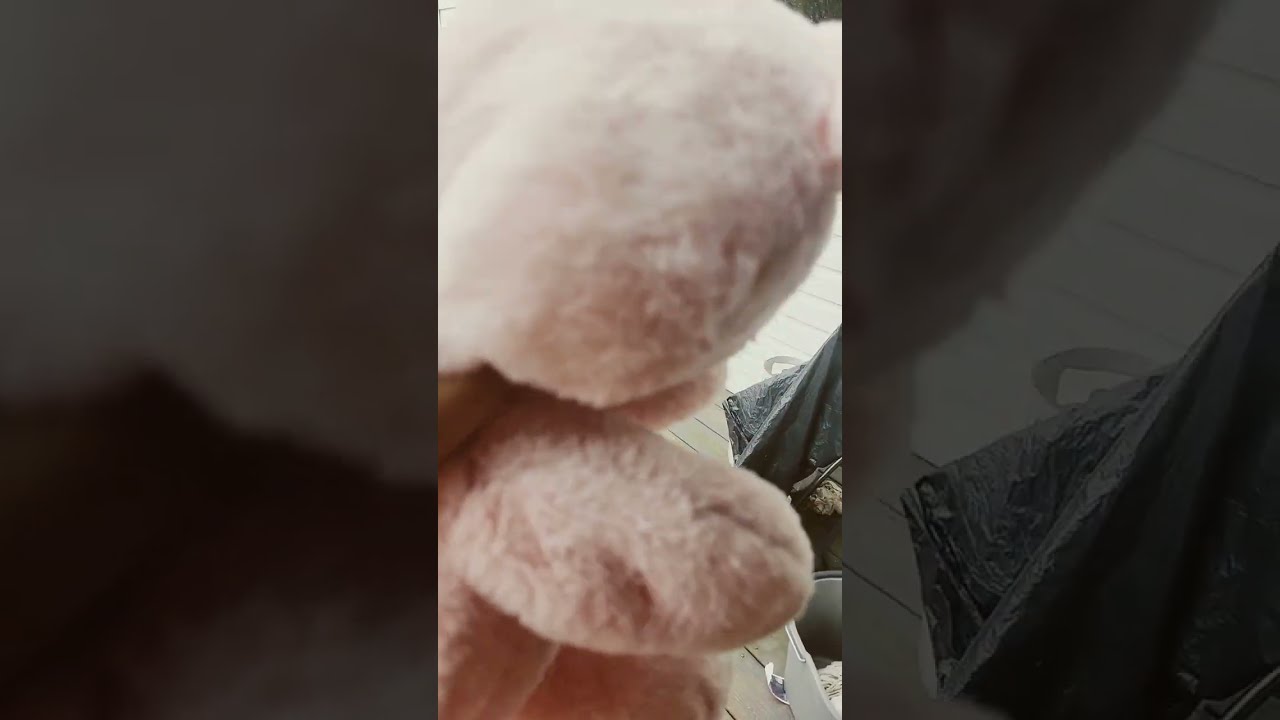The image depicts a close-up of a pink teddy bear facing to the right, with its head slightly pointed down and its right paw resting on what seems to be an outdoor wooden deck, possibly simulated wood with greenish hues visible. The teddy bear's fur features bright highlights towards the left top of its head, creating a mix of illuminated and shaded areas. The middle third of the image, both horizontally and vertically, is occupied by the central figure of the teddy bear while the rest of the image serves as the background. Interestingly, the same teddy bear's head is repeated in the background, blown up and dimmed with a dark filter, making it more difficult to discern. This filtered background extends from top to bottom and is split into two sections, occupying the left and right thirds of the image. Additional details in the background include what appears to be white wooden planks, a black plastic bag with a white handle, and potentially a hand holding the teddy bear by the neck on the far left, giving a hint of human presence. Overall, the photograph presents a multi-layered and detailed composition of the teddy bear against a rough, possibly outdoor setting.